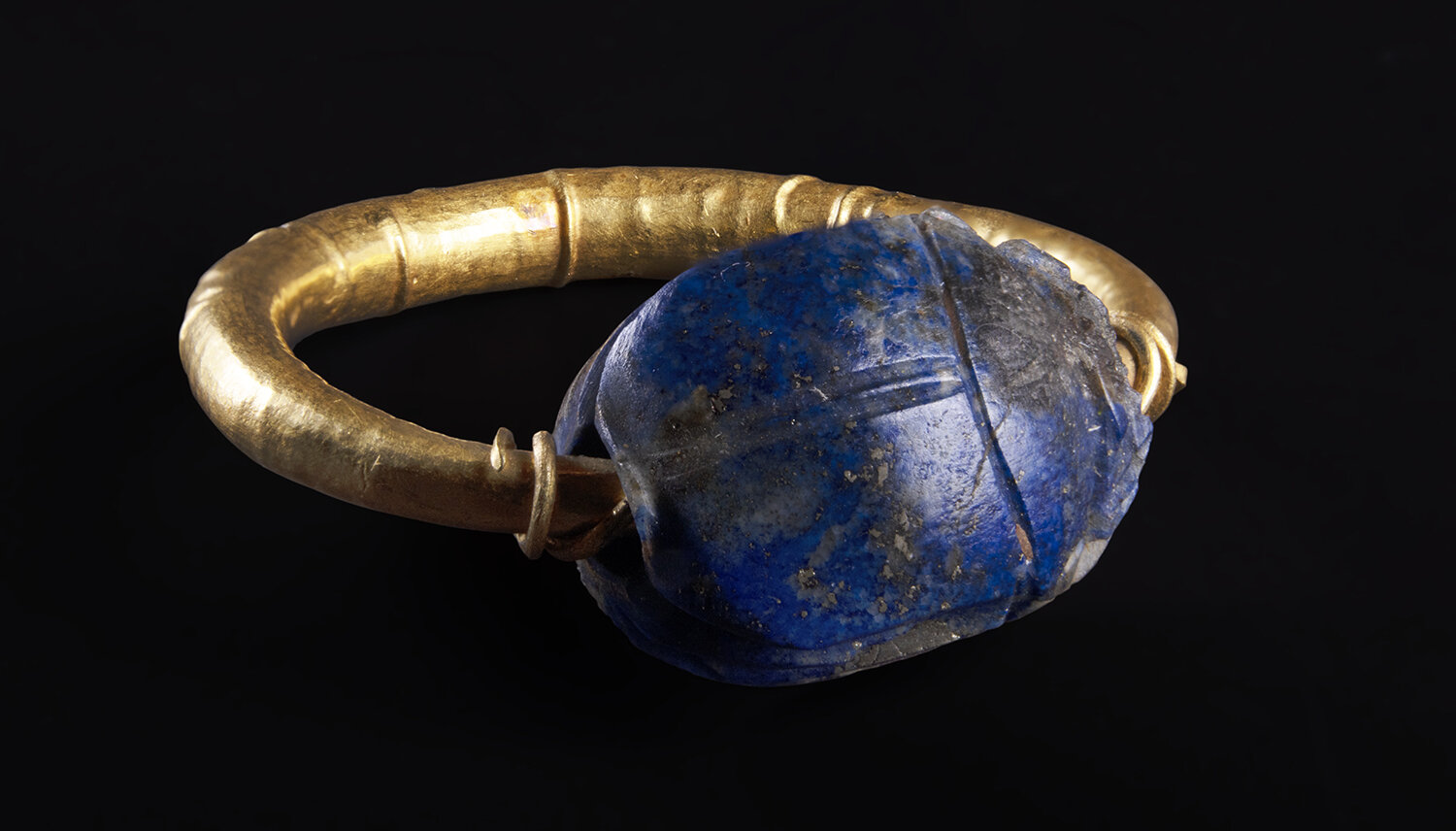Displaying prominently against a stark black background, the relic in the image is an intricately handcrafted piece of ancient jewelry, most likely a bracelet given its size and form. Made from a polished gold or gold-tinted metal, possibly bronze or copper, the oval-shaped artifact features a distinctive design adorned with ripples and rings along its band, narrowing towards an elaborate central embellishment. This central feature is an aged, vibrant blue stone, resembling a scarab—an emblem often associated with Egyptian art and symbolizing protection or rebirth. The stone, although not shiny, has historical allure given its rich color and detailed beetle-like carving, suggesting great antiquity. The artifact shows signs of age with noticeable brown stains or rust, indicative of its historical journey through time.